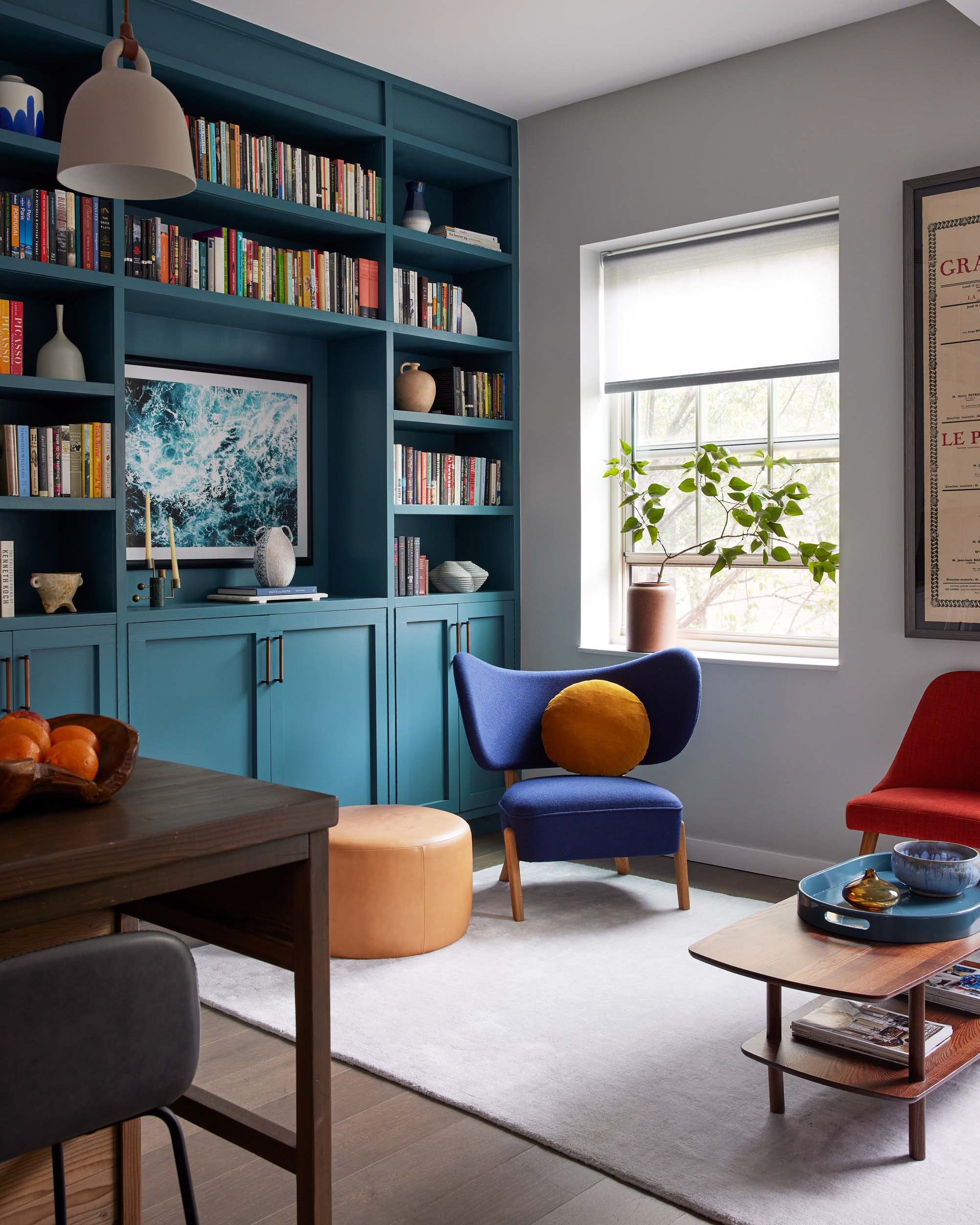The image depicts a cozy and eclectic living room that doubles as a dining area. On the lower left, a polished dark brown wooden table supports a bowl filled with vibrant oranges, hinting at its dual function. Adjacent to this, there's a sleek black chair. The room is characterized by its dark hardwood floors, partly covered by a short, white rug. A curved, cushioned blue chair with light wooden legs and an orange sun-shaped throw pillow rests on the rug. Nearby, on the right, a red chair stands in front of a small, brown wooden coffee table adorned with various decorative elements. The right wall is white and features a window with a white frame, partly opened, allowing a potted plant with green leaves to bask in the natural light. A poster is also seen on this wall.

Dominating the left side of the room is a tall, teal-colored shelving unit filled with books and vases, with cabinet doors at the bottom for additional storage. Among the items on the shelves is a framed picture, possibly depicting ocean waves. Above, on the upper left, a unique hanging light fixture shaped like a giant white coffee mug adds a whimsical touch to the space. The ceiling is white and slightly curved. Completing the scene is a small backless peach-colored chair and a secondary light brown wooden table with a shiny blue platter, adding further layers to this richly detailed living area.